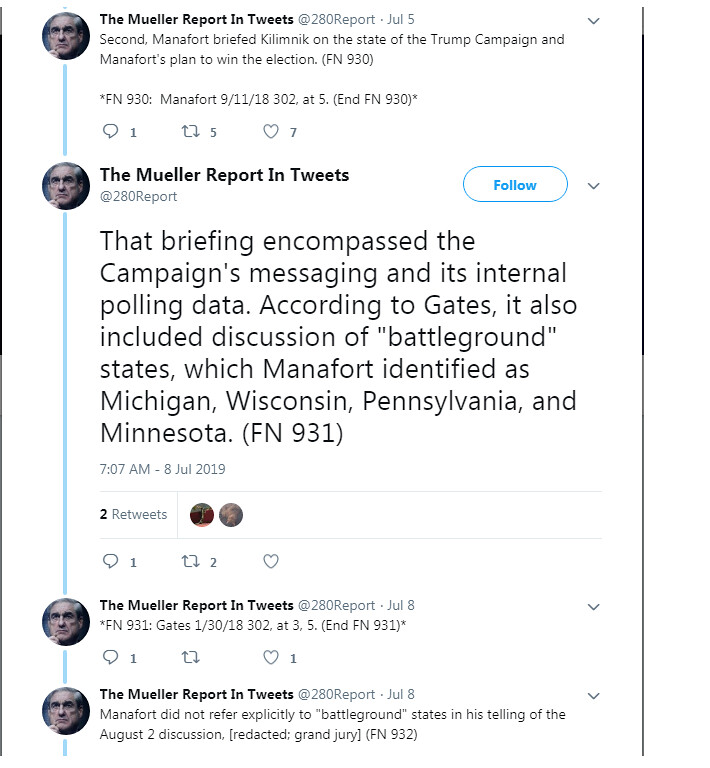The image depicts a tweet thread from a Twitter account named "The Mueller Report in Tweets," posted on July 5th. It appears on a cell phone screen. The tweets detail key information from the Mueller report, specifically focusing on Paul Manafort's actions. In one tweet, it states that "Manafort briefed Kilimnick on the state of the Trump campaign and Manafort's plan to win the election" (FN 930). The thread continues, noting that the briefing covered the campaign's messaging, internal polling data, and discussions of battleground states, including Michigan, Wisconsin, Pennsylvania, and Minnesota, according to Gates. Additionally, the thread mentions that Manafort did not explicitly refer to battleground states during his recounting of the August 2 discussion, with a portion of the text redacted for the grand jury. The image also includes a picture of Mueller.